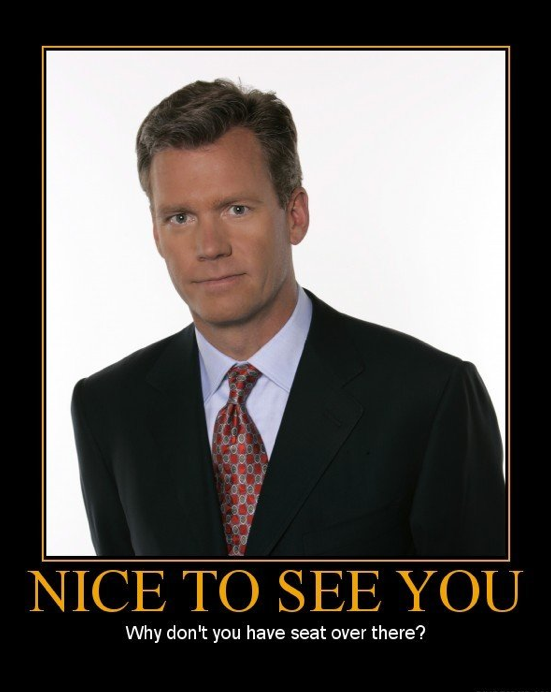This image is a horizontally aligned rectangle photograph set within a black frame. The bottom side of the black frame is thicker than the left and right sides, which are themselves thicker than the top side. Inside the black frame is a thin yellow line, forming another parallel rectangle within the outer rectangle. The image itself has a white background with no additional elements or special lighting.

The focal point of the image features Chris Hansen, a well-known talk show host. Hansen is a Caucasian man with short, neatly styled brown hair combed back from his forehead, adding volume. His complexion is slightly tanned, and his appearance suggests he might be wearing some light foundation makeup. He is dressed in a black suit jacket over a white collared shirt and a predominantly red checkered tie with white and possibly black patterns. Hansen's expression is serious as he looks directly at the camera. He is posed slightly off-center to the viewer's left, making only his left ear partially visible and more of his right ear.

Below the photograph, within the lower section of the yellow-lined frame, there is text. The first line reads "NICE TO SEE YOU" in all-caps yellow font reminiscent of Times New Roman. Centered beneath that, in smaller white font that looks like Comic Sans and has only the 'W' capitalized, it says "Why don't you have a seat over there." This caption is a nod to Hansen's television show "To Catch a Predator," where he would confront individuals engaging in sexually explicit conversations with decoys posing as minors.